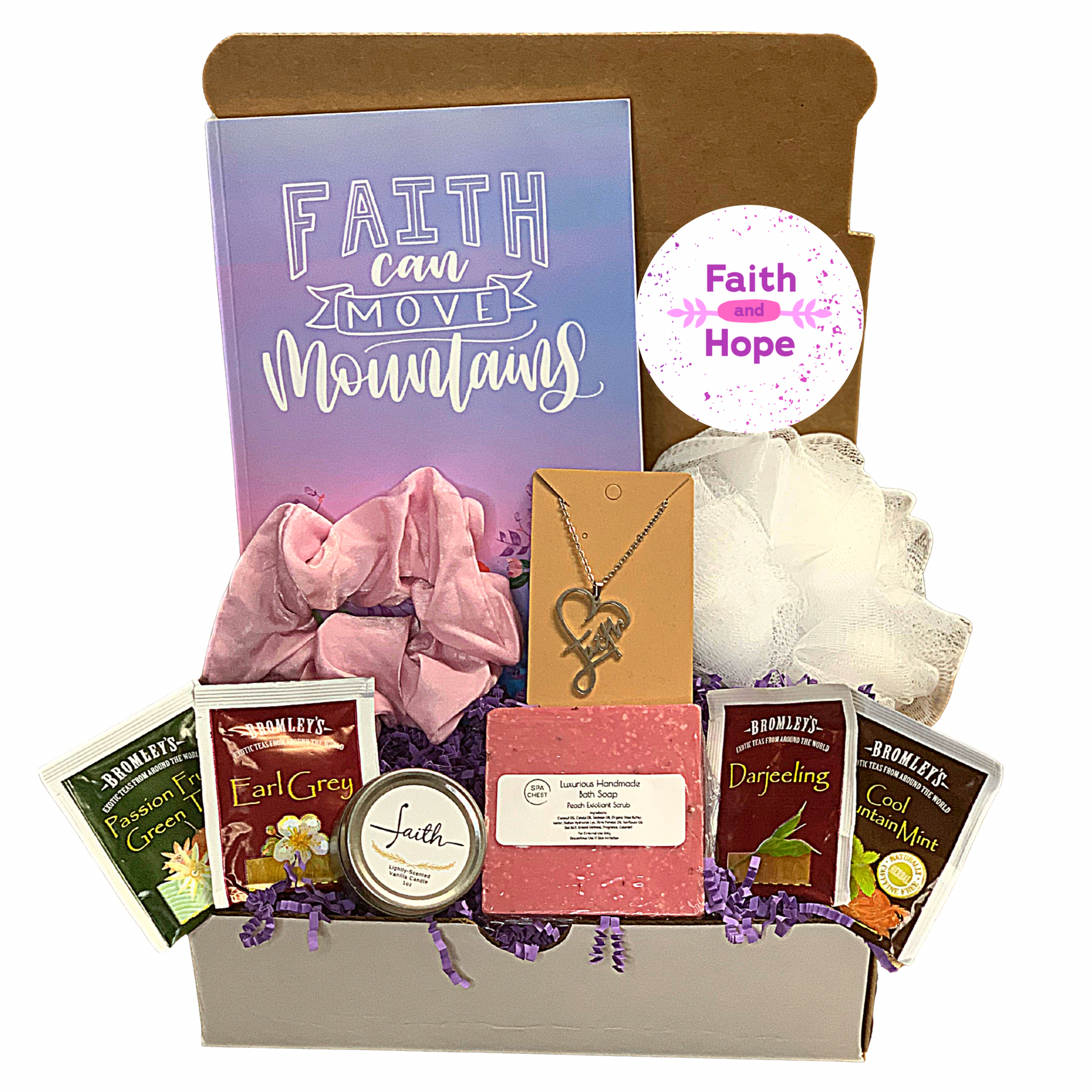This photograph features an open gift basket, set against a white background, with contents meticulously arranged and visible. The open cardboard box, brimming with purple confetti paper, prominently displays a variety of items. In the background, a card with white text on a purple gradient reads "Faith Can Move Mountains." A round sticker with the words "Faith and Hope" in purple and pink lettering adds a decorative touch to the scene.

The gift basket contains an assortment of teas, including Earl Grey, Passion Fruit Green Tea, Darjeeling, and Cool Mountain Mint, each packaged in distinctively colored sachets. Alongside the teas, there is a handmade square bath soap, a bath loofah, a hair scrunchie, and a small, round tin labeled "Faith Cream." A gold heart necklace with a pendant engraved with the word "Faith" adds a touch of elegance, while a piece of pink fabric, resembling either a scrunchie or decorative cloth, is also included.

Overall, the basket's thoughtful arrangement and varied contents, framed by a supportive and inspiring message, make it an appealing and heartfelt gift.